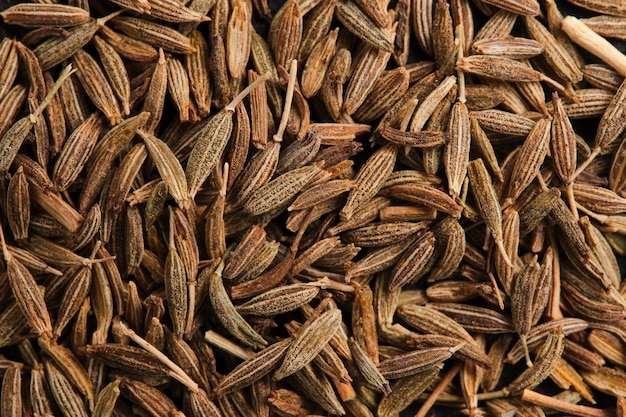The photograph captures a close-up view of a dense pile of long, ridged seeds that bear a strong resemblance to fennel seeds. These seeds are scattered in various directions, creating a layered effect that completely covers the entire image space. They display muted shades of browns and tans, adding a natural, earthy tone to the scene. Some of the seeds feature stems, while others appear to be broken, indicative of their dried state. The arrangement of hundreds of seeds in the picture suggests they may have fallen en masse from a tree during a seasonal bloom. Notably, there is a small white stick in the bottom left corner, which stands out due to its brightness against the otherwise uniform seed background. The overall composition has a somewhat artistic quality, with not a single area left uncovered by the seeds, save for some shadows creating darker spots amidst the layers.